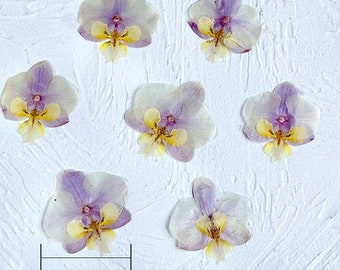This photograph captures a meticulously arranged display of seven flat-pressed pansy flowers set against a textured white background, reminiscent of plaster or a textured wall. Each pansy features petals in subtle shades of pastel purple, yellow, and white. The flowers, positioned equidistantly, form a circular design with six surrounding one central bloom. There is some gray shadowing within the background texture, contributing to the overall muted and soft aesthetic of the image. Notably, in the lower left corner of the photograph, a grayscale measurement bar is visible, though it lacks numerical markers. Two of the flowers at the top edge appear slightly cropped, adding a touch of dynamism to the composition.